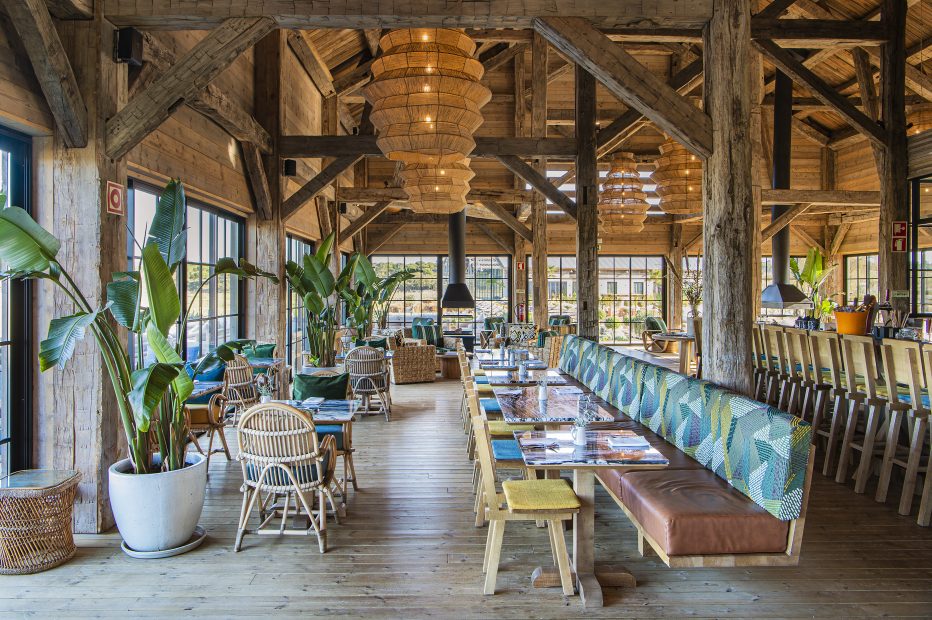This image depicts an expansive, rustic-style restaurant interior designed to evoke a beachy, barn-like atmosphere with a casual dining environment. The space, which can accommodate around 60 diners, features a variety of seating arrangements including long benches with tables, wicker chairs along tall, wide windows, and solitary chairs opposite tables. The ceiling showcases exposed wooden beams and is adorned with log rafters, accentuated by Japanese lantern-style light fixtures and candelabra-like woven material. A cozy bar area seats at least 10 patrons on bar stools. The restaurant incorporates natural elements with numerous large tropical plants in substantial pots strategically placed around the windows and doors, adding a fresh, vibrant touch to the rustic charm. Additionally, there are two fire pits with chimneys, enhancing the warm and inviting ambiance of the space.